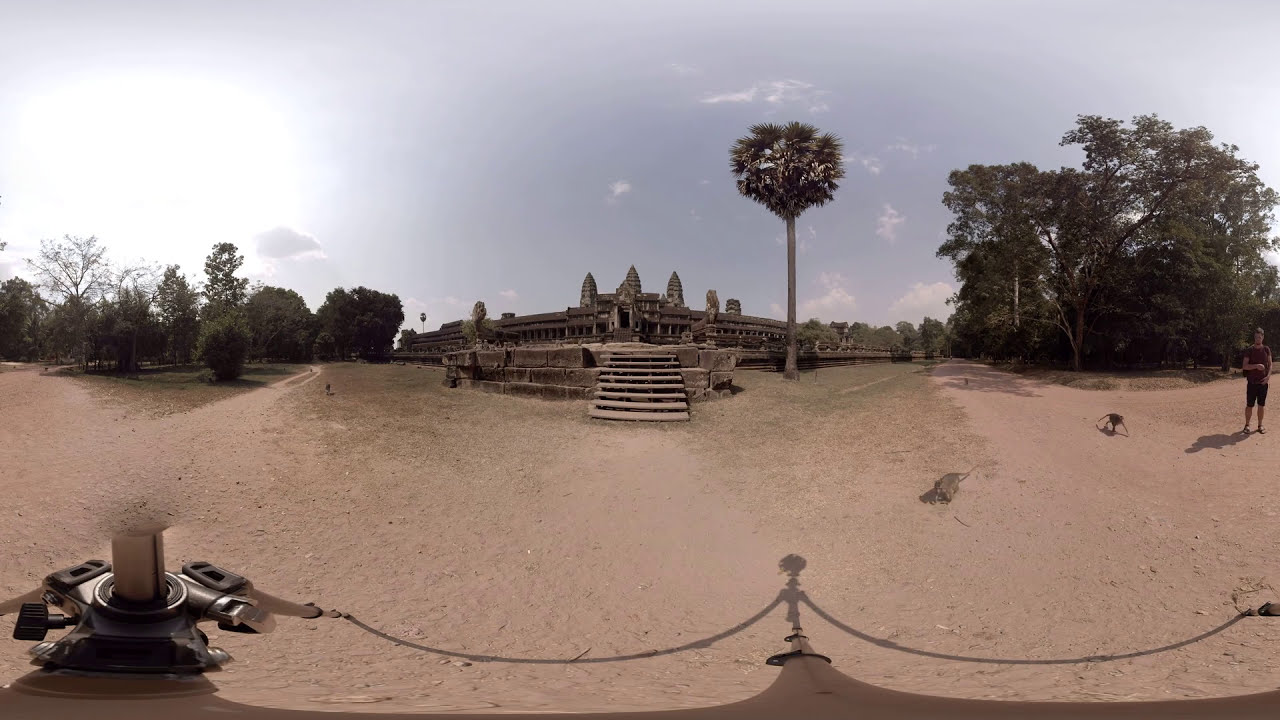The photograph captures a panoramic view of a vast and ancient stone temple, likely from Southeast Asia, surrounded by a sandy landscape with sporadic patches of grass. The central feature is a large, weathered, gray-stone structure with towering, rectangular pillars that taper to points at the top, indicative of a bygone era. Steps composed of substantial stone bricks lead from the bottom center of the image up to the temple entrance, which in itself is a testament to ancient craftsmanship. Two small brown monkeys can be spotted near a person standing to the right of the temple, alongside a tall, slender palm tree. Additional trees frame the photograph from both sides. The presence of some camera or fencing equipment with ropes and metal parts is visible along the bottom edge of the distorted, fisheye-styled image taken on a bright, sunny day. The photograph exudes an air of antiquity and timelessness with its intricate stonework and weathered surfaces.